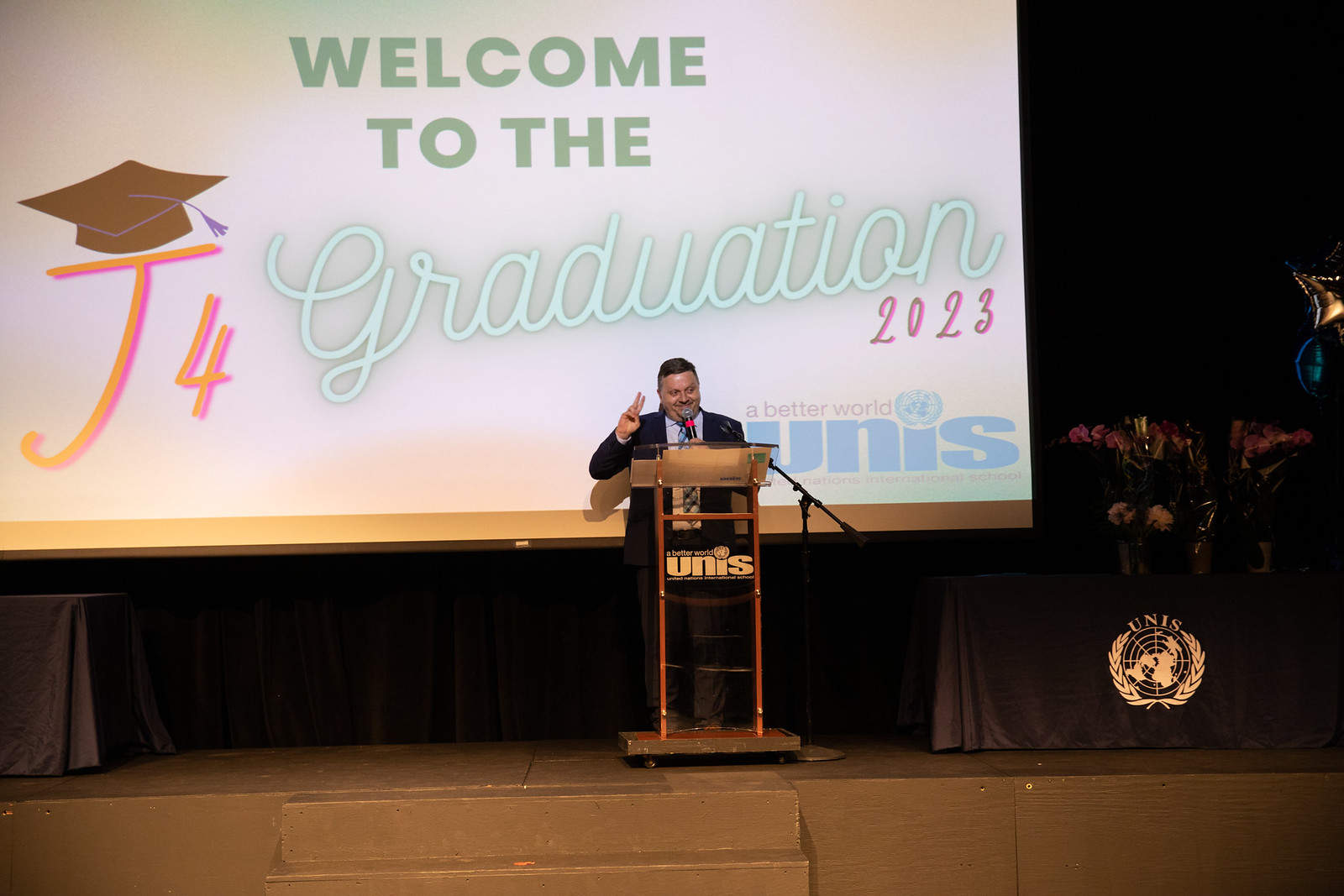In this detailed image, a speaker is addressing an audience at a graduation ceremony held on a stage with brown steps leading up to it. The speaker, a heavyset man with short brown hair, is dressed in a black suit, white collared shirt, and blue plaid tie. He stands behind a wooden podium with a glass top and glass front, which is about five feet tall. The podium features the text "A Better World UNIS" and the logo of the United Nations International School.

Behind the speaker is a pull-down screen displaying a presentation with the text "Welcome to the J4 Graduation 2023," where "Welcome to the" is capitalized in green. The text has a white interior, giving it a neon appearance. Above the letters "J4," there is an illustration of a graduation cap. The dark stage background is complemented by a black tablecloth-covered table with the UNIS logo, which includes a gold circumference of a globe flanked by olive branches. The table is adorned with flowers, adding a touch of elegance to the scene. This detailed setting emphasizes the importance and formality of the graduation event at the United Nations International School.